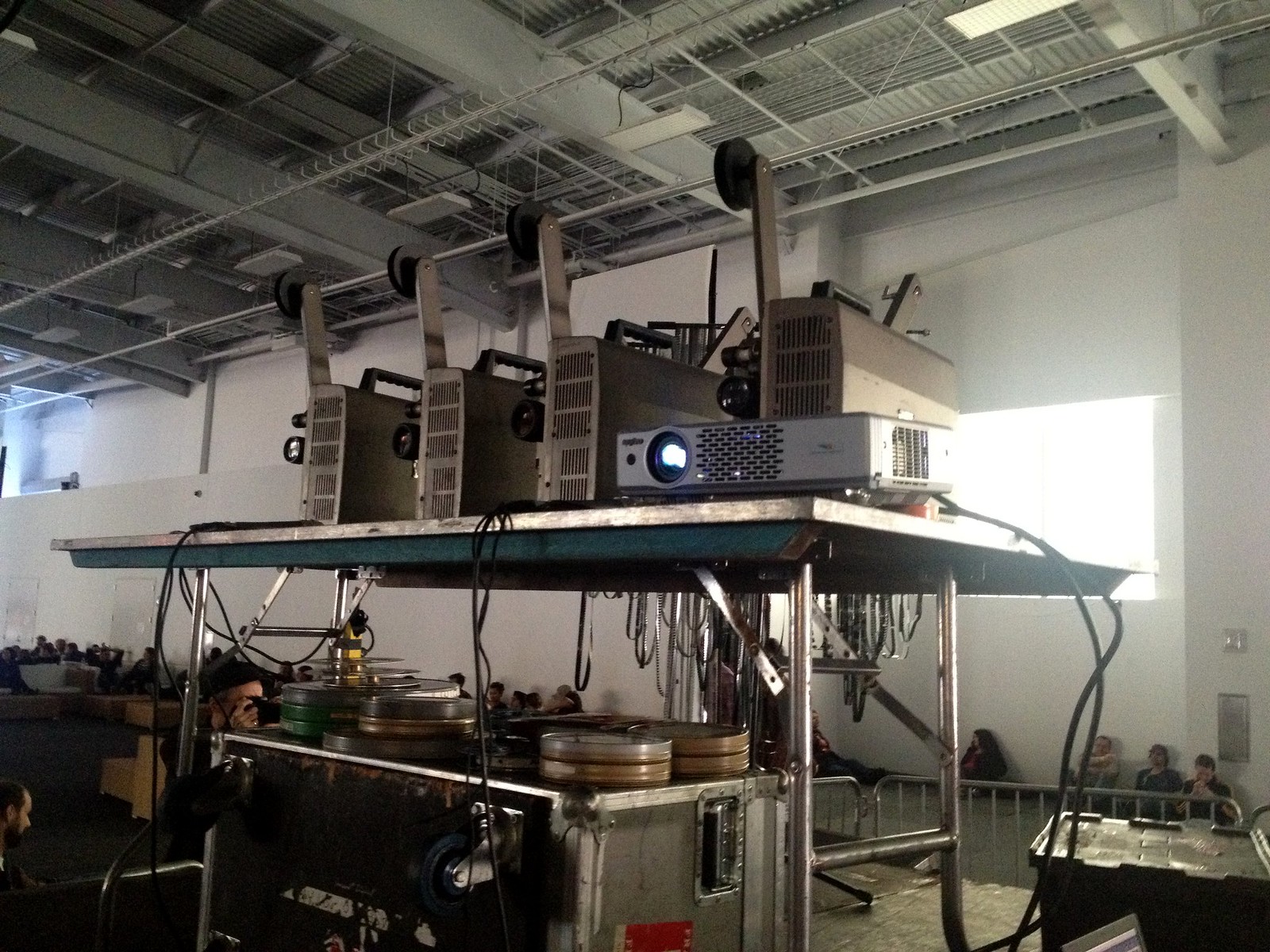The photograph appears to be taken inside an industrial warehouse or garage with a white back wall and a gray ceiling supported by metal beams. Dominating the center of the image is a folding table with a silver edge and legs. Atop the table are five vintage film projectors, with one distinct projector actively in use. Beneath the table sits a cart filled with numerous film reel containers and loose film cascading off the sides. The right side of the cart also holds a dark-colored plastic container, and nearby, a large silver box with circular disks on top is visible. The foreground includes a person whose face is partially obscured by a metal instrument, while their hand is prominently seen. Background elements include people sitting against the wall – possibly taking a break or watching a film – and another individual entering from the left. The top of the image features industrial lighting and ceiling grating, enhancing the warehouse atmosphere.